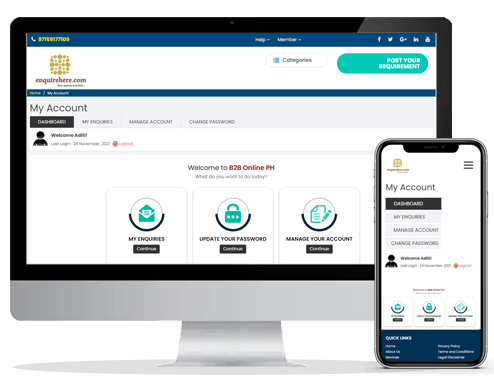This image features an advertisement showcasing a website's compatibility across desktop and mobile devices. The website displayed appears to be "enquirehere.com". A distinct, gold-colored, square-shaped symbol adorned with dots is positioned in the upper left corner of the site. On the left side of the image, there is a sophisticated desktop monitor with a silver and black frame. To its right, a sleek silver mobile phone mirrors the desktop content. 

The desktop screen sports a clean, white background with a prominent green button in the upper right corner. The user is currently viewing the "My Account" section, featuring tabs such as "My Inquiries", "Update Your Password", and "Manage Your Account". This section is titled "Welcome to 828 Online PH". 

The mobile device displays the same account section and tabs, albeit in a layout optimized for smaller screens, ensuring ease of access and navigation on mobile platforms.